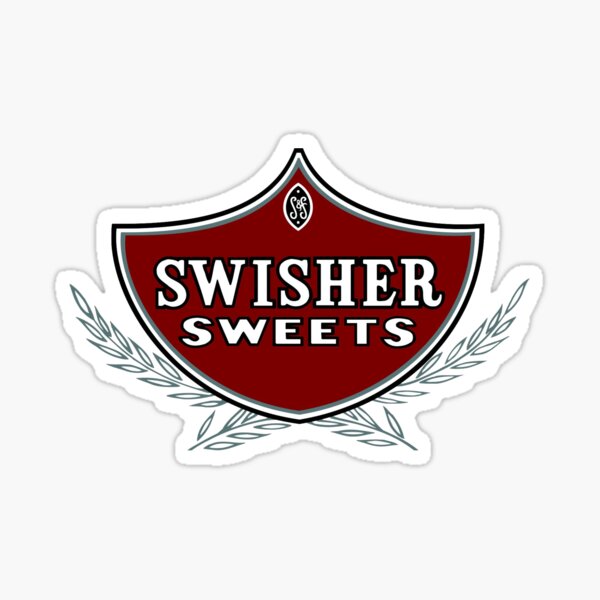This image features the distinct logo of Swisher Sweets, a well-known brand of cigars. Central to the picture is an oxblood red shield-shaped emblem with bold, white capital letters spelling "Swisher Sweets." The shield has a traditional coat-of-arms design with a U-shaped curve at the bottom and two upward curving lines meeting at the top, reminiscent of a classic war shield. This emblem also incorporates stylized leaves or feathers on either side, adding an intricate decorative element. The entire logo is centrally positioned on a plain white background, enhancing its visibility and prominence. The white text and detailed emblem create a strong contrast against the deep red backdrop, making the Swisher Sweets logo easily recognizable and strikingly vivid.